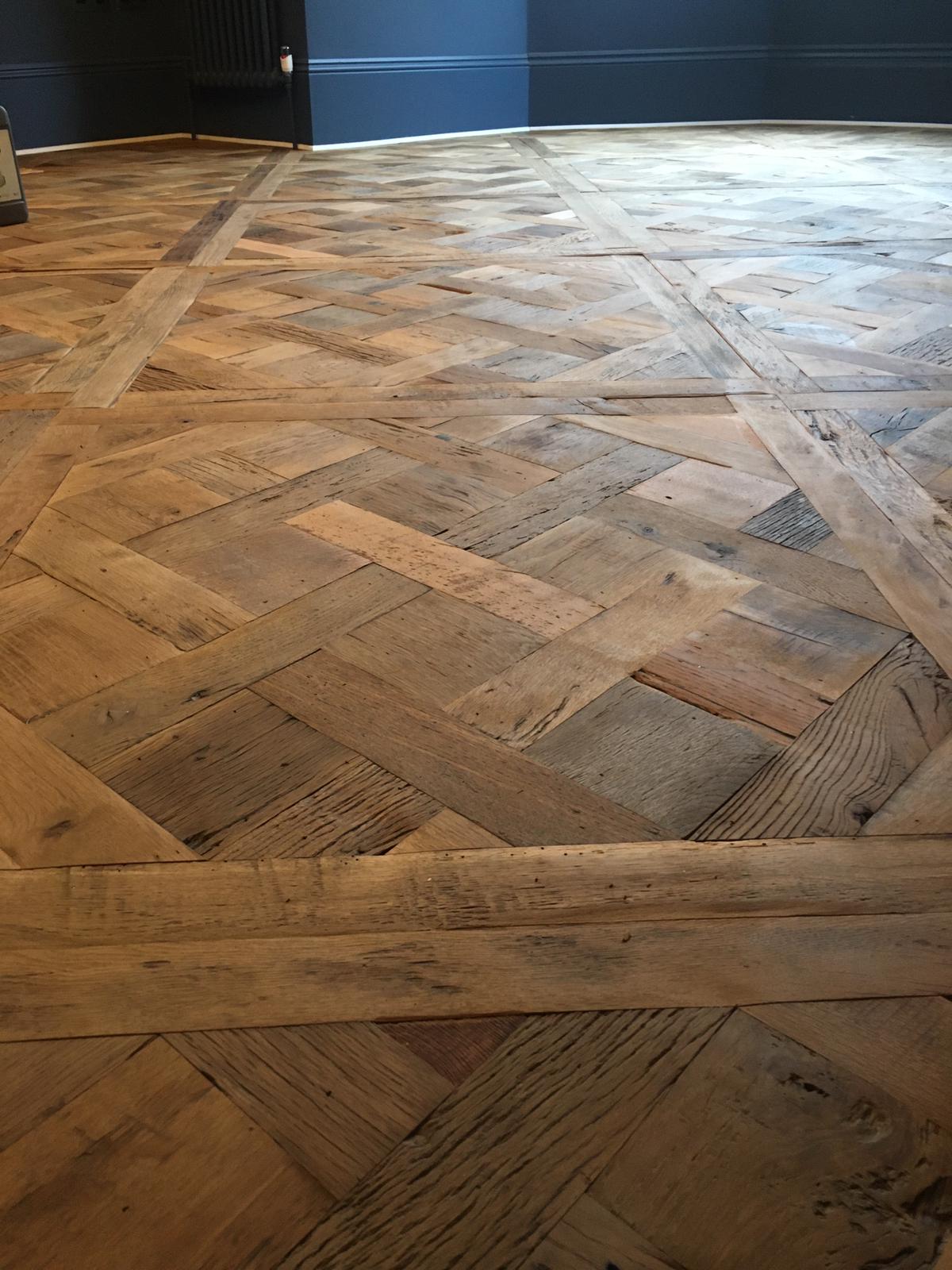This image depicts a wooden floor characterized by a crosshatch or crisscross pattern, with wooden panels woven into each other and delineated by square outlines. The floor, a mix of light and dark brown hues, shows signs of wear and tear, including scuff marks and some color fading over time. The wooden surface, which extends almost the full length of the image, appears uneven, potentially warped and slightly moist, resembling a long tabletop or expansive flooring that could be mistaken for a dance floor.

In the background, there is a wall painted in dark blue with a horizontal strip of light blue and white running through it. The wall features two small white lines and what may be a doorknob or door lock. On the left side of the image, there is a heating apparatus or heater, partially visible, alongside a small stand-up sign resting on the wooden surface. The scene is bright, with natural sunlight indicating it's daytime, illuminating the interior space.